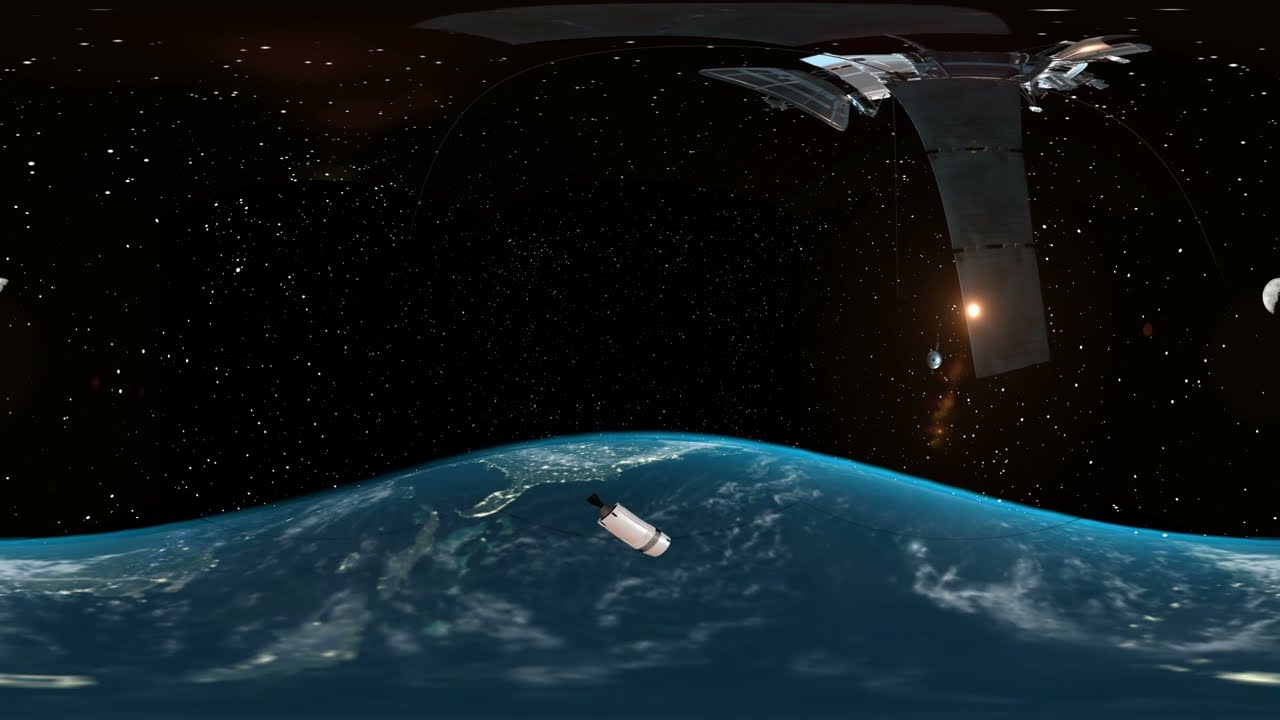The image depicts a computer-generated scene of outer space, viewed through a fisheye lens, likely from a satellite or the International Space Station. In the foreground, a distorted, wave-like representation of Earth is visible, with Florida and the ocean's lights distinctly discernible. Blurry white clouds obscure parts of this blue, mountainous terrain. A white, cylindrical metal object with a black tail — reminiscent of a message in a bottle — floats directly in front of the Earth. Above, the blackness of space is peppered with white dots representing stars. A complex black satellite with a dangling component and a blazing light on its left edge hovers overhead. To the right, a partial view of a planet, likely the moon, adds depth. Another round, silver satellite appears in the background beyond the dangling object. Near the top right corner of the frame, another satellite is visible, targeted by a red laser beam on one of its solar panels, showcasing Rayleigh scattering.